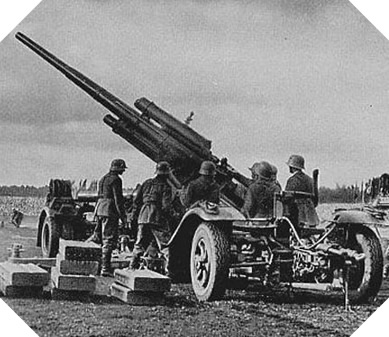This vintage black-and-white photograph, with its diagonally clipped corners reminiscent of an old scrapbook, captures a scene from what appears to be World War I. The focus is a large, cannon-like anti-aircraft artillery gun, mounted on a vehicle chassis with large wheels. The long black barrel of the gun is directed towards the upper left corner of the image. Surrounding the gun are five soldiers in early 1900s military uniforms, complete with helmets, jackets, trousers, and boots, distinguishing their attire as circa 1917-1918. These men, standing in a semicircle, are intently facing the base of the artillery, engaged in their task. To the left side of the photograph lie three stacks of ammunition boxes, likely containing munitions for the gun. The background reveals a grassy field, extending to a horizon marked by a line of trees beneath a gray, cloudy sky. The image, dominated by shades of gray, black, and light gray, encapsulates a poignant moment from the wartime era.